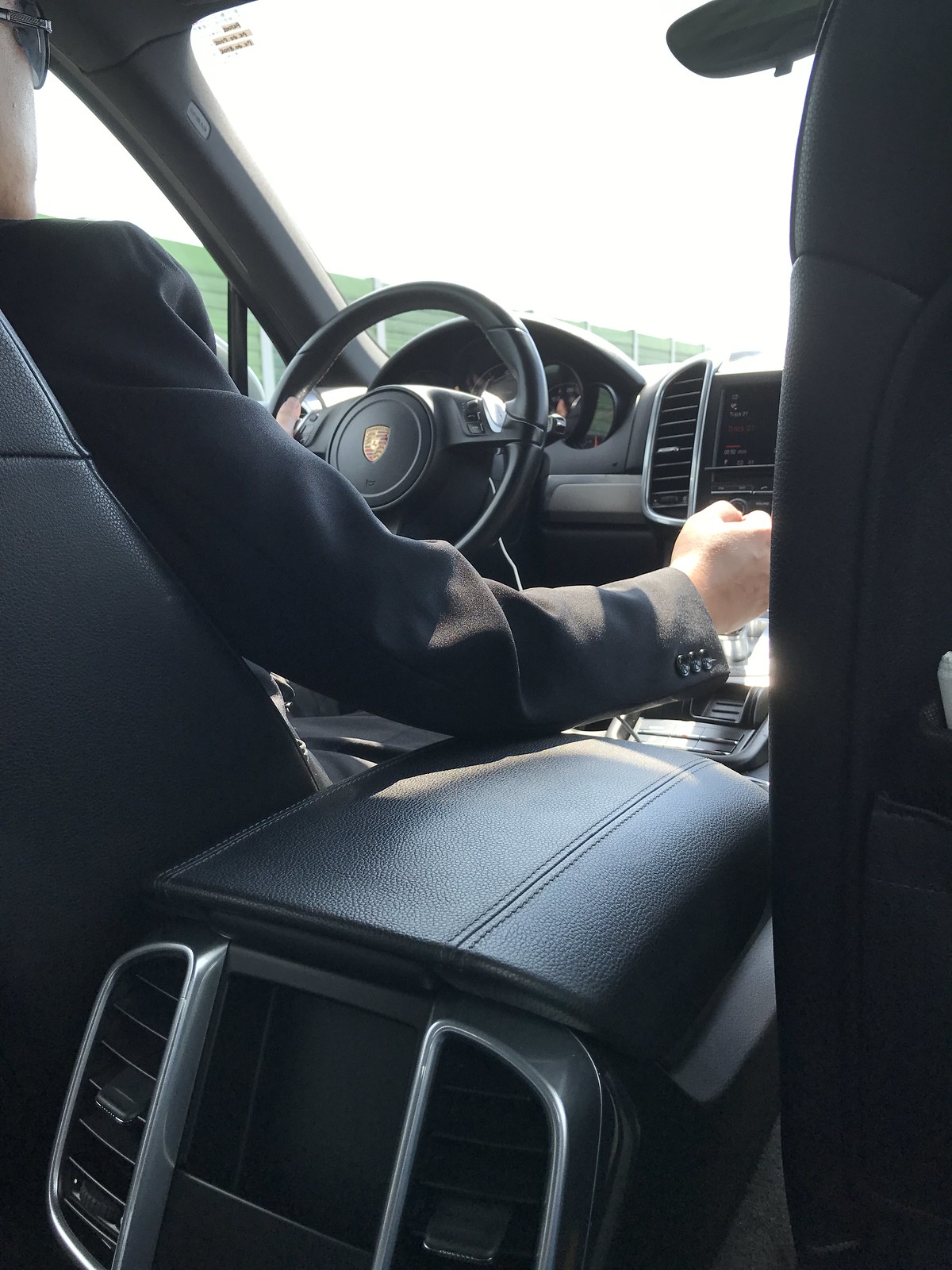The photograph captures a scene from the backseat of a sleek car, most likely a Lamborghini, as suggested by the emblem on the steering wheel. The car's interior is predominantly black, with the driver’s seat occupied by a white male adorned in a black suit jacket, complete with three-buttoned sleeves. The man, who is also wearing black sunglasses, has his right hand poised on the gearstick, showcasing a firm grip indicative of controlling the vehicle. The image showcases several interior details: the speedometer, though hard to read, the dashboard, the AC vent, the media display, and a part of the rearview mirror. Sunlight filters in, highlighting the bright yet cloudy sky visible through the front windshield. The view outside reveals a green building along with the hints of a green field or meadow, adding a touch of nature to the otherwise modern and dark interior. The picture is evidently taken during the daytime, with the photographer positioned on the back right-hand seat.